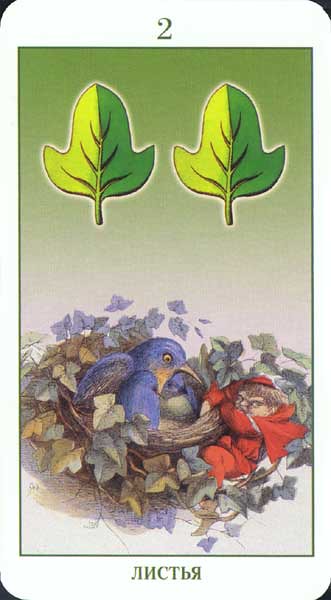The image appears to be an illustration reminiscent of a playing card or a tarot card. At the top, a green numeral "2" is prominently displayed. At the bottom, there is green text in Russian, consisting of six letters, though its meaning is unclear. The central portion of the illustration, shaped like a rectangle that is taller than it is wide, may represent one side of a card.

A green border frames the entire image, and two green leaves adorn the top. The background features a gradient that transitions from a deep forest green at the top through lighter shades, ultimately blending into a white hue with a hint of purple.

In the lower part of the image, a bluebird is depicted in a nest, surrounded by ivy. Nearby, a small, sinister-looking person dressed in red clings to the edge of the branch. This figure, smaller than the bird, is looking to the right with a wary expression. The bird, positioned on the left, glares at the human figure. The person's red attire, including a cap resembling those worn in the Catholic Church, billows in the wind. The overall scene suggests a potential layer of political commentary.